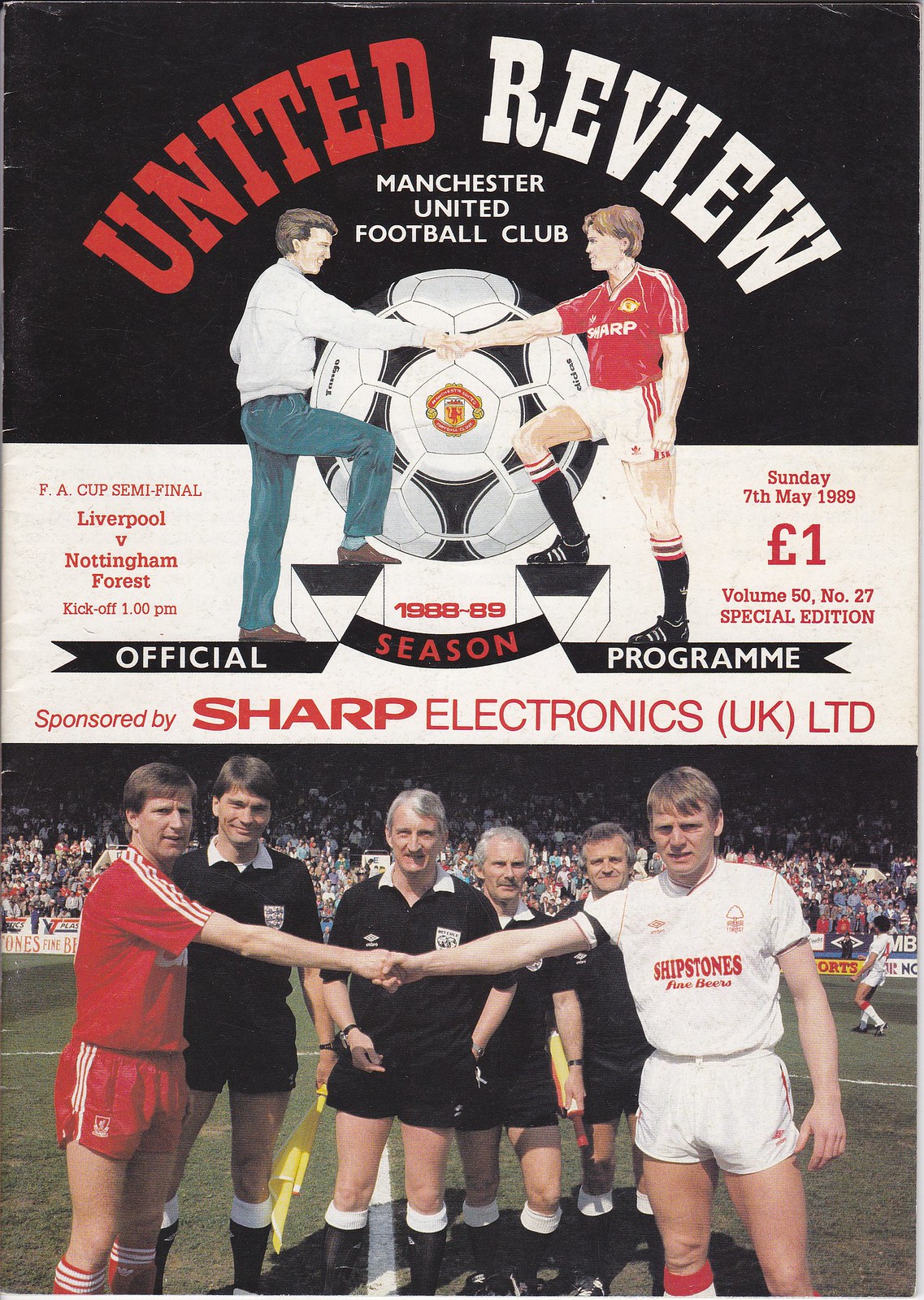This image is a detailed poster for the Manchester United Football Club's official program for the 1988-89 FA Cup semifinal between Liverpool and Nottingham Forest. Dominating the top section, a black box displays "United" in bold red text, alongside "Review" and "Manchester United Football Club" in white. Below this, a central illustration features a person in a white sweater and blue jeans shaking hands with a soccer player dressed in a red shirt, white shorts, black socks, and black sneakers. The player's shirt is prominently branded with "Sharp" on the front. They shake hands in front of a giant soccer ball adorned with the Manchester United logo. The white section beneath the illustration provides event details in red and black text. It reads "FA Cup Semi-final Liverpool versus Nottingham Forest, kick-off 1 p.m. Sunday, 7th May 1989, one pound, volume 15, number 27, special edition," and notes sponsorship by Sharp Electronics UK Limited. At the bottom, a photograph depicts two soccer players, one in red and the other in white, shaking hands, accompanied by four officials in black and white uniforms standing behind them.